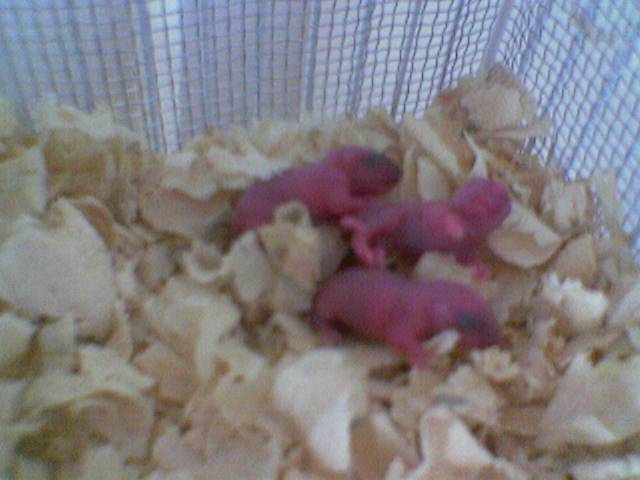This is a very out-of-focus and grainy photograph capturing a corner of a cage that appears to contain freshly born baby rodents, possibly hamsters or mice. The cage itself features a fine wire exterior, possibly metal screening or wire with plastic coating, designed with very small squares suitable for such tiny animals. The bottom of the cage is lined with a thick bed of large wood shavings, resembling curled pine bedding typically used in rodent habitats. The image prominently showcases the three or four shockingly pink and purple, nearly translucent, baby rodents. Their eyes are not yet open, indicating their very young age. These tiny creatures are lying in a small pile on the bedding, with one appearing to have its legs slightly raised as if it had been moving. The wood shavings dominate most of the photo, leaving the baby rodents grouped towards the center and upper right, adding to the composition's overall blurry and indistinct quality.